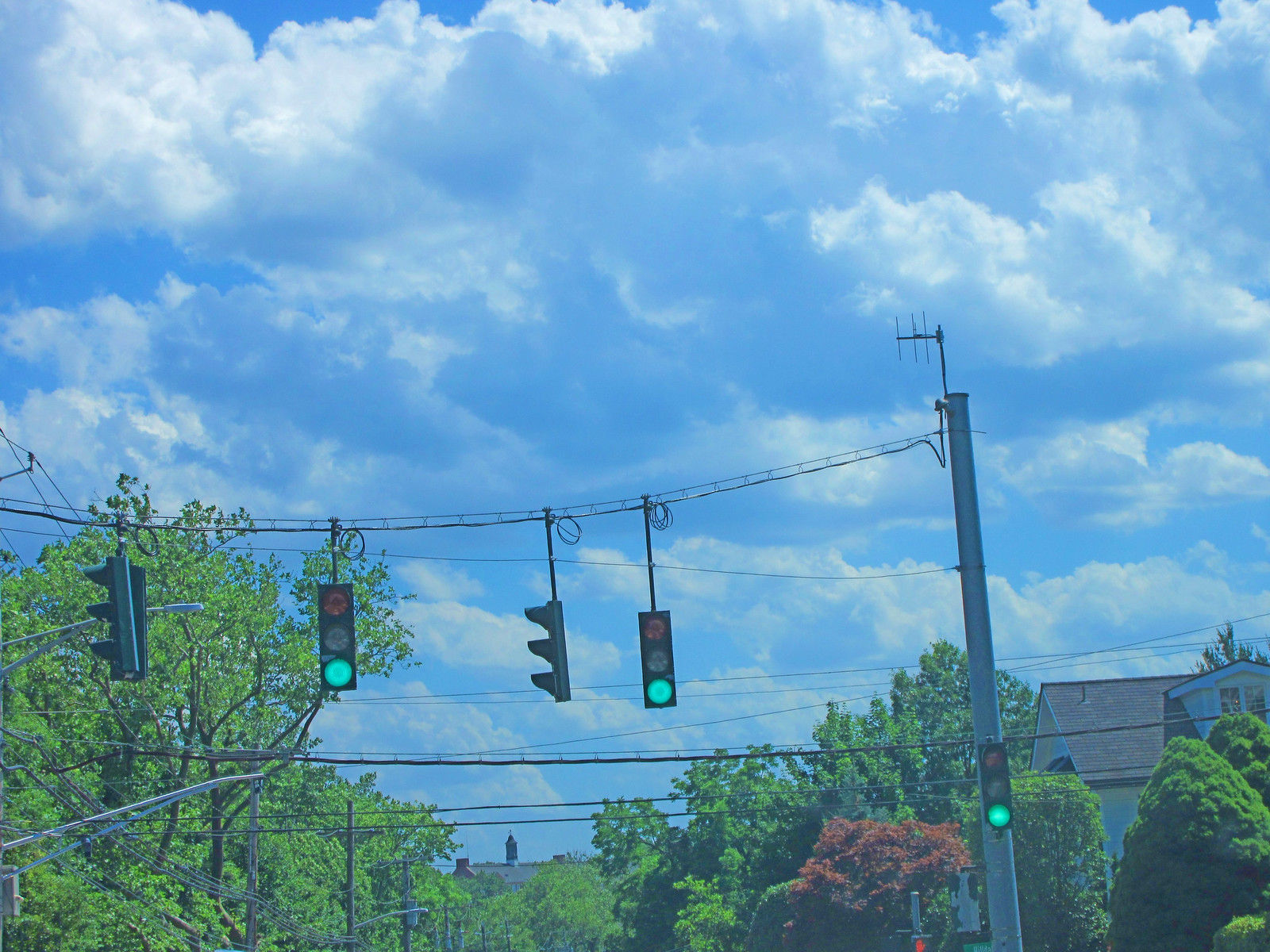In this out-of-focus photograph, we see a close-up, zoomed-in view from the perspective of someone sitting in a car, looking up at a complex traffic signal installation at an intersection. Four traffic lights hang from a wire strung between two large, round poles. Two of these lights face directly towards the viewer, showing green signals, while the other two face left, likely intended for cross traffic. At the top of one pole, a small Yagi antenna is attached, with several wires extending from it. Additionally, a smaller traffic light hangs from the wire below, also displaying a green signal. In the background, the sky is filled with puffy white and blue-gray clouds, providing a picturesque backdrop. On the right side, the tops of trees and a house with a black roof and white trim are visible. Electrical, telephone, and cable wires crisscross the scene, adding to the urban complexity. This detailed view captures the multi-directional signaling at a busy intersection, framed by the serene sky and surrounding neighborhood greenery.